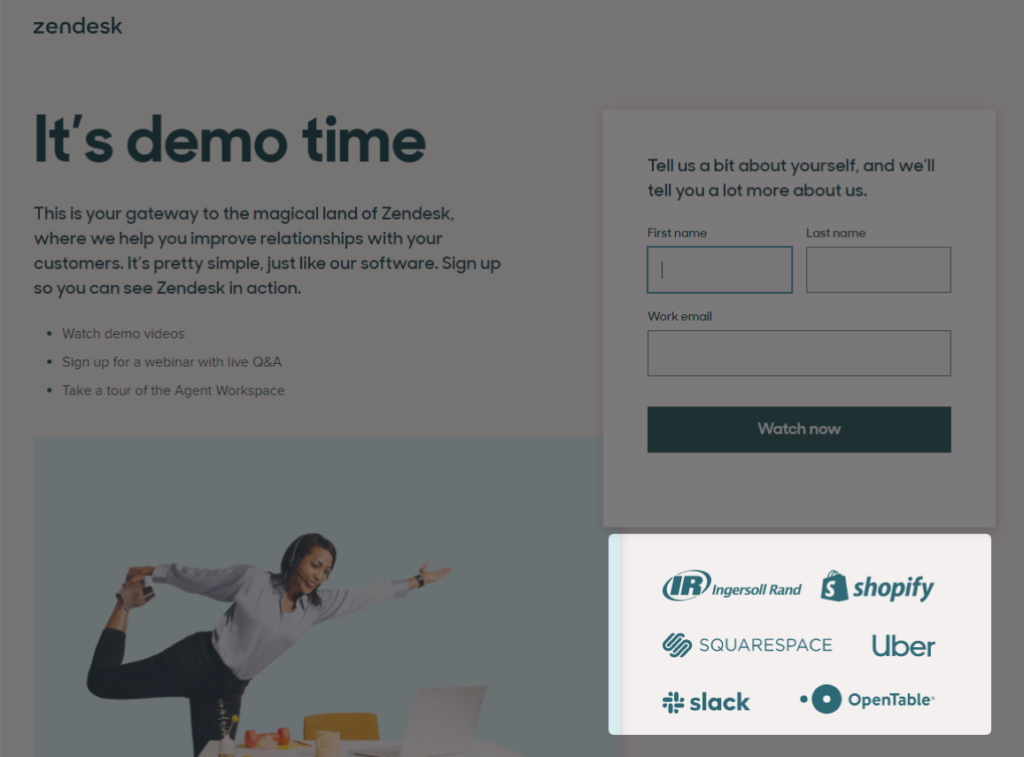A cropped screenshot from the Zendesk website showcases a clean, white background, prominently featuring the Zendesk logo in the top left corner. Below the logo, a bold blue banner reads, "It's demo time," introducing the rest of the text which states, "This is your gateway to the magical lands of Zendesk where we help you improve relationships with your customers. It's pretty simple, just like our software, sign up so you can see Zendesk in action."

This introductory text is followed by three vertical bullet points providing options to:
1. Watch demo videos.
2. Sign up for a webinar with live Q&A.
3. Take a tour of the agent workspace.

Directly beneath this section, there is a square image depicting a woman leaning over a desk in a playful manner.

On the right side of the screenshot, a large white square contains a heading that says, "Tell us a bit about yourself and we'll tell you a lot more about us." Following this, there are input boxes for "Name," "Last Name," and "Work Email." At the bottom of this white section, a smaller square showcases various company logos against a bright white background.

The remainder of the screen has a dark overlay, similar to the effect when a pop-up is activated, dimming the background to focus attention on the central content.